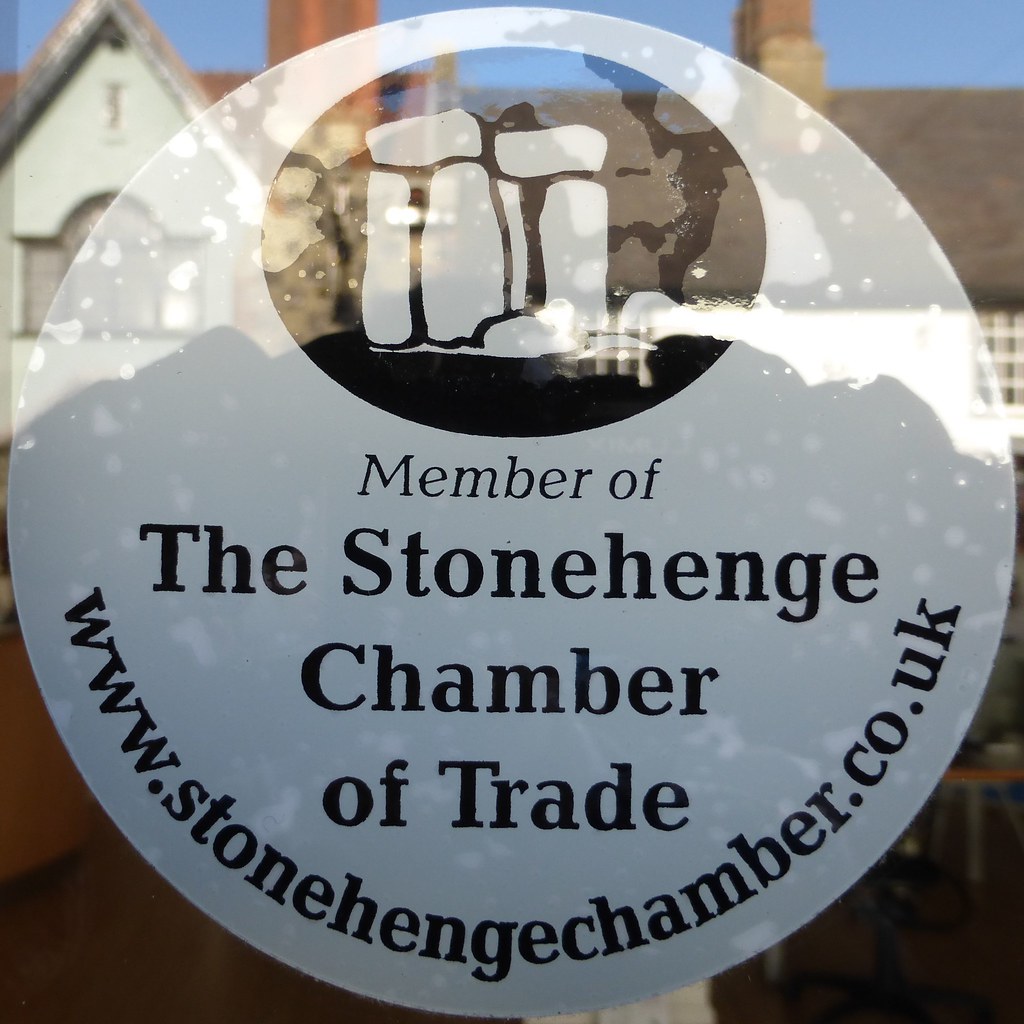The image features a circular logo prominently displayed on a glass window. The logo occupies the upper third of the circle with a smaller circle containing a stylized depiction of Stonehenge, etched to look like two stones. Below this image, the text reads "Member of the Stonehenge Chamber of Trade" and curves along the bottom of the logo is the website "www.stonehengechamber.co.uk". The signage appears to be taped on the inside of the glass, as small air pockets are visible. In the background, through the glass, a quaint cottage with a pointed roof is visible. The cottage features two chimneys that extend the width of the roof, an arched doorway on the left, and a window with small square panes on the right side. Dark grey areas are visible in the bottom right of the background, enhancing the contrast and historic charm of the scene.